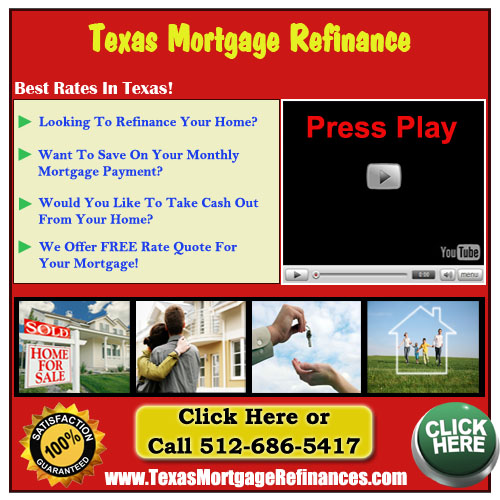The advertisement features a vibrant red background with prominent yellow text at the top stating, "Texas Mortgage Refinance." Directly below, in bold white letters, it reads, "Best Rates in Texas!" On the left side, there's a tan box with four green bullet points outlined in blue text, each addressing key mortgage refinance benefits: "Looking to refinance your home?", "Save on your monthly mortgage payments", "Take cash out from your home", and "We offer free rate quotes for your mortgage." On the right, there's a black box featuring a silver play button, resembling a YouTube video interface, with text advising to "Press Play."

Below these main sections are four images: a "Home Sold" sign in front of a house, a joyful couple embracing, a hand passing house keys to another hand, and a family playing on a lawn with an outlined image of a house around them. At the bottom of the flyer, it instructs, "Click here or call 512-686-5417," accompanied by a website link, www.texas-mortgage-refinances.com, and concludes with a satisfaction guarantee emblem.